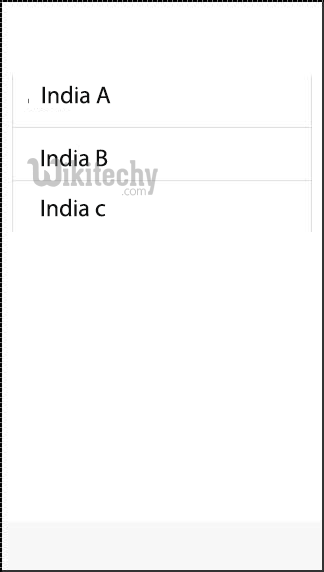The image appears to be a carefully edited screenshot from a smartphone. The top area, which typically contains the timestamp and other status icons, has been cropped out, leaving a clean, white background. A light gray bar spans the bottom 10% of the image, providing a subtle contrast to the otherwise white background. This white background is framed by a solid black border that encompasses the entire image.

At the center of the image are three distinct lines of text. The first line reads "India A" with a capital 'A', rendered in black font. Directly beneath it, the second line displays "India B," also with a capital 'B' and in black font. The third line presents "India c," with a lowercase 'c', staying consistent in black font.

The background beneath these textual elements is unclear, but it seems to be plain white, as if the words were directly superimposed onto it. On the upper left-hand side of the image, there are two short horizontal lines stacked vertically. Each horizontal line terminates with a short vertical line, creating rectangular shapes or cells, seemingly designed to contain the text "India A," "India B," and "India c".